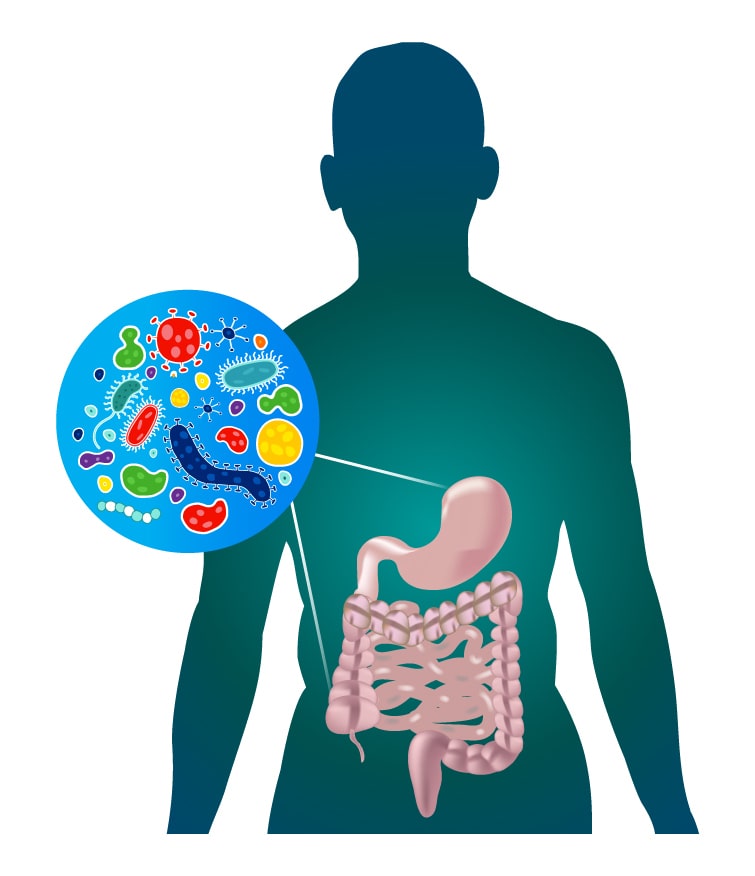This detailed digital diagram, likely from a textbook, features a silhouette of the human body with a gradient color scheme transitioning from dark green at the bottom to light greenish-blue towards the middle, and darker at the top. Inside the silhouette, a detailed depiction of the digestive system is highlighted in pink, showing the stomach at the top, followed by the coiled small intestine and the large intestine wrapping around it. The image cuts off around the wrist level of the silhouette. To the left of the silhouette, there is a prominent blue circle filled with variously shaped and colored microorganisms, representing different bacteria and germs in red, purple, yellow, green, and white. This circle has two white lines, or arrows, emanating from it, pointing towards the stomach and the large intestine, illustrating their connection to the microbiome. The overall background of the image is blue, enhancing the visibility of the detailed elements.